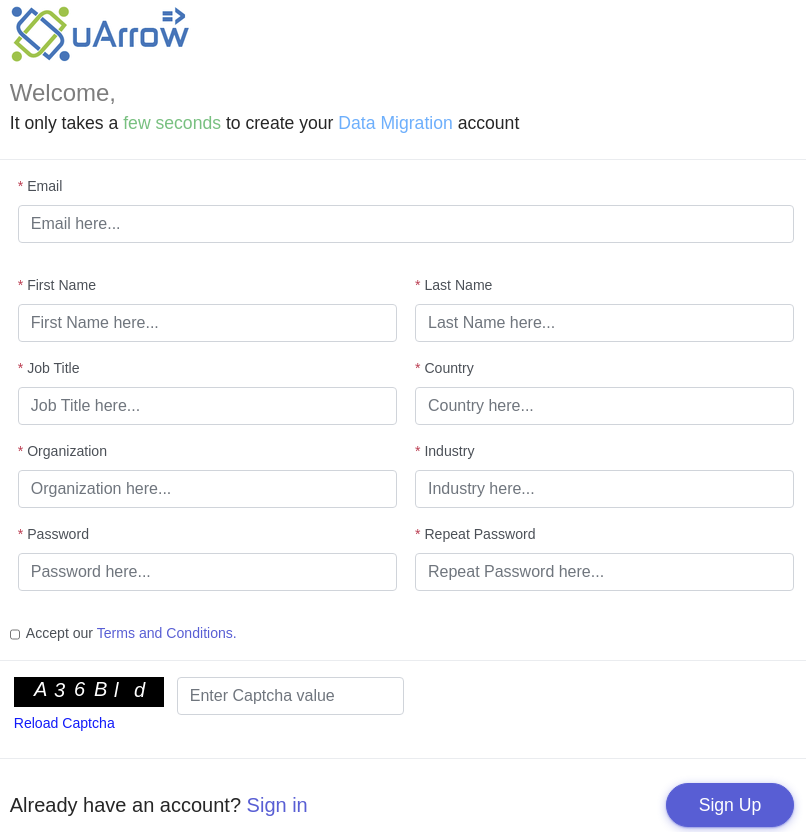This image displays a Data Migration program interface. The logo located at the top left is composed of green and blue colors and includes an insignia that is spelled either as "UARR" or has an arrow instead of "R" indicating "WU arrow". Directly below the logo, the word "Welcome" is prominently displayed, followed by a concise statement: "It only takes a few seconds to create your Data Migration account."

The form fields presented are sequential as follows:
1. **Email**: An input box labeled for entering your email address.
2. **First Name**: An input box labeled for entering your first name.
3. **Last Name**: An input box labeled for entering your last name.
4. **Job Title**: An input box labeled for entering your job title.
5. **Country**: An input box labeled 'Country here' for specifying your country.
6. **Organization**: An input box labeled 'Organization here' for specifying your organization.
7. **Industry**: An input box labeled 'Industry here' for specifying your industry.
8. **Password**: An input box labeled 'Password here' for entering your password.
9. **Repeat Password**: An input box labeled 'Repeat Password here' for confirming your password.

Additionally, there is a checkbox for accepting the terms and conditions, with "terms and conditions" hyperlinked in purple text. Below this checkbox, there is a CAPTCHA entry prompt displaying "A36BID", with an option to reload the CAPTCHA. 

At the bottom of the screen, on the left side, there's a text prompt "Already have an account? Sign in," and on the bottom right, there is an option to "Sign Up".